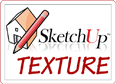This is a top-down photograph of a road or pavement area, predominantly gray with white highlights, possibly representing concrete or asphalt. A distinctive feature of the image is a narrow strip of grass running straight down the center. The grass varies in condition, with some tufts being bright green while others appear dried and brown, scattered around the edges. Rocks are sporadically scattered amidst the grass. In the top left and bottom right corners, there is a rudimentary logo depicting a house and a pencil alongside text that reads "SketchUpTextureClub.com." The logo is associated with the website www.sketchuptextureclub.com, and it indicates that this is a free downloadable texture, likely intended for use in architectural visualization projects. The layout dimensions of the image suggest that it is wider than it is tall, approximately in a 3:1 ratio.